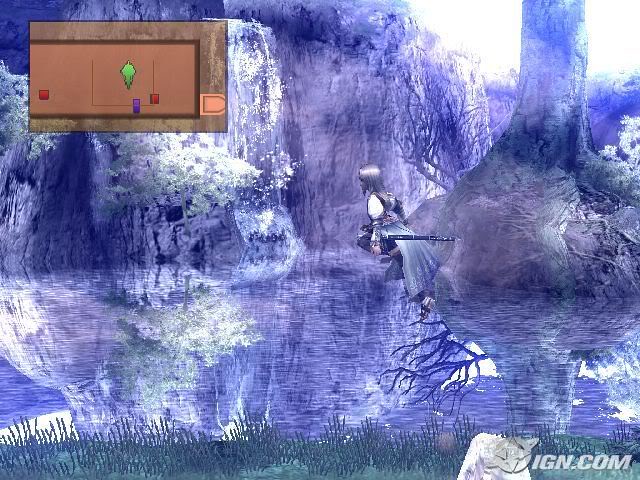The image features detailed elements characteristic of a video game scene. In the bottom right corner, the watermark "IGN.com" is visible. Dominantly in the center, a green character is present, surrounded by vivid environmental elements. The top left corner hosts a rectangular element. The bottom section of the image contains the words "We're Blue," followed by a red dot.

The central part of the image bursts with colors and activity. The scene is set against a lush backdrop of trees and bushes positioned on the left side, with water reflecting these natural elements at the bottom. A character, who appears to be dynamically jumping or walking across the water, adds to the action. The character is distinguishable by their flowing skirt, a sword in a scabbard, a white poofy shoulder, and long blue hair.

The rocky and grassy terrain at the very bottom left reflects the leafy structure of a mountainside, further enhancing the natural, adventurous ambiance of the scene.